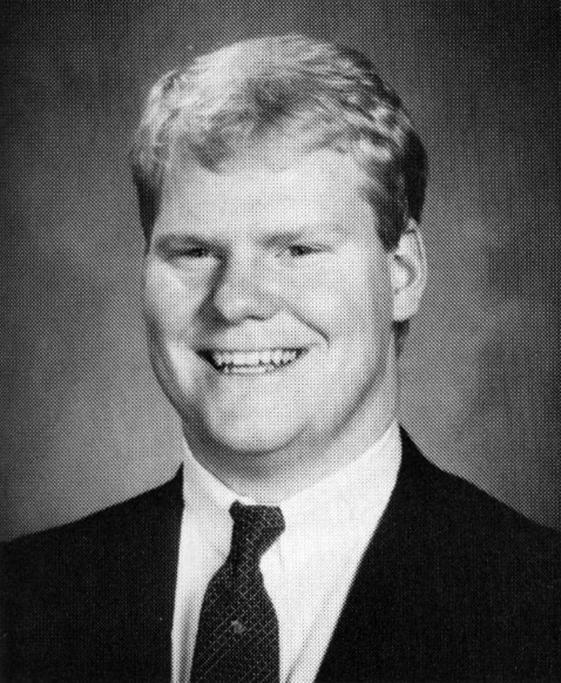This black-and-white photograph, reminiscent of a vintage yearbook photo, features a young, clean-shaven white man in a formal attire. He is wearing a dark suit jacket, a white shirt buttoned to the top, and a diagonally checkered tie. The man, who has short blonde to brown hair parted on the side, is smiling warmly, with eyes that also convey a sense of happiness. His smile reveals his pointy white teeth. He is slightly angled away from the camera while looking directly at it, adding a dynamic quality to his pose. The photograph, with its gray background and focus on the man's face and shoulders, carries an air of professionalism perhaps hinting at a studio setting.